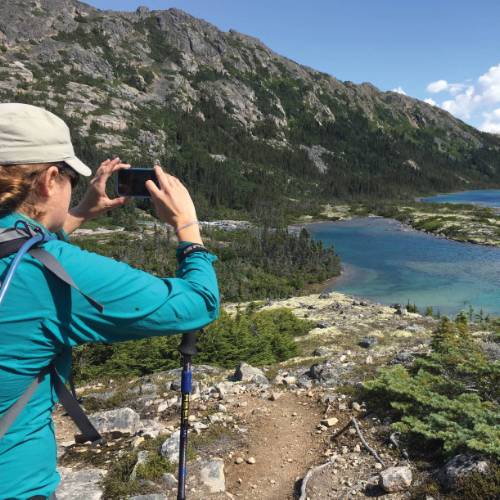In this vibrant outdoor photograph, a person captured in the act of photographing a stunning landscape dominates the left side and bottom left corner of the frame. The individual, visible from the waist upwards and facing away from the camera, is dressed in a long sleeve blue shirt, a gray cap, and bears a black strap backpack equipped with a blue hydration tube. Their right wrist is adorned with a black strap attached to a hiking pole, indicating they are likely on a hiking trip. The person is using a square-shaped smartphone to take a picture of the expansive scene in front of them.

The landscape is a breathtaking tapestry of nature, featuring a large, bright blue lake nestled at the base of a rugged gray and white mountain. The mountain, adorned with various trees and vegetation, rises majestically under a clear, light blue sky dotted with occasional white clouds. Patches of tan dirt interspersed with small gray rocks and green vegetation stretch out in the foreground. Bathed in sunlight, the entire scene exudes a sense of serenity and natural beauty, illustrating a picture-perfect moment in a picturesque setting.